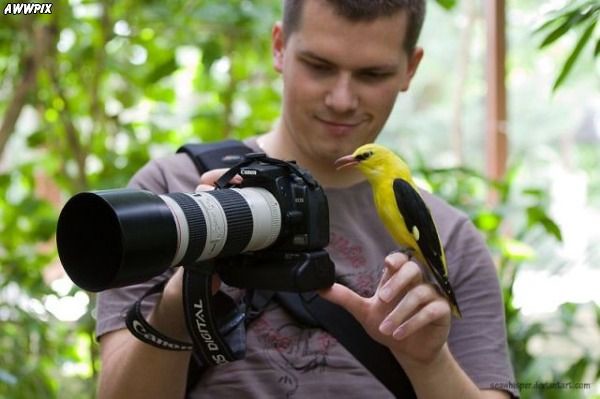In this charming photograph, a young white male with short brown hair and a gray t-shirt featuring a silkscreened pattern stands in a lush, tropical setting. He holds a black camera with an impressive black-and-white telephoto lens in his right hand, his camera strap resting on his shoulder. His left hand is extended, with a beautiful yellow tropical bird perched on his index finger. The bird, adorned with black wings, medium-length orange beak, and black markings around its eyes, contrasts strikingly with the foliage. The man's expression is a captivating blend of amusement and smirk as he gazes at the bird. The background is a blurred mix of green leaves, small tree branches, and light filtering through, suggesting a jungle or atrium environment. In the upper left-hand corner, the letters "A-W-W-P-I-X" are visible, while the lower right-hand corner contains partially legible text resembling a website, "schweizer something dot com." The overall scene radiates a serene and endearing moment in nature photography.